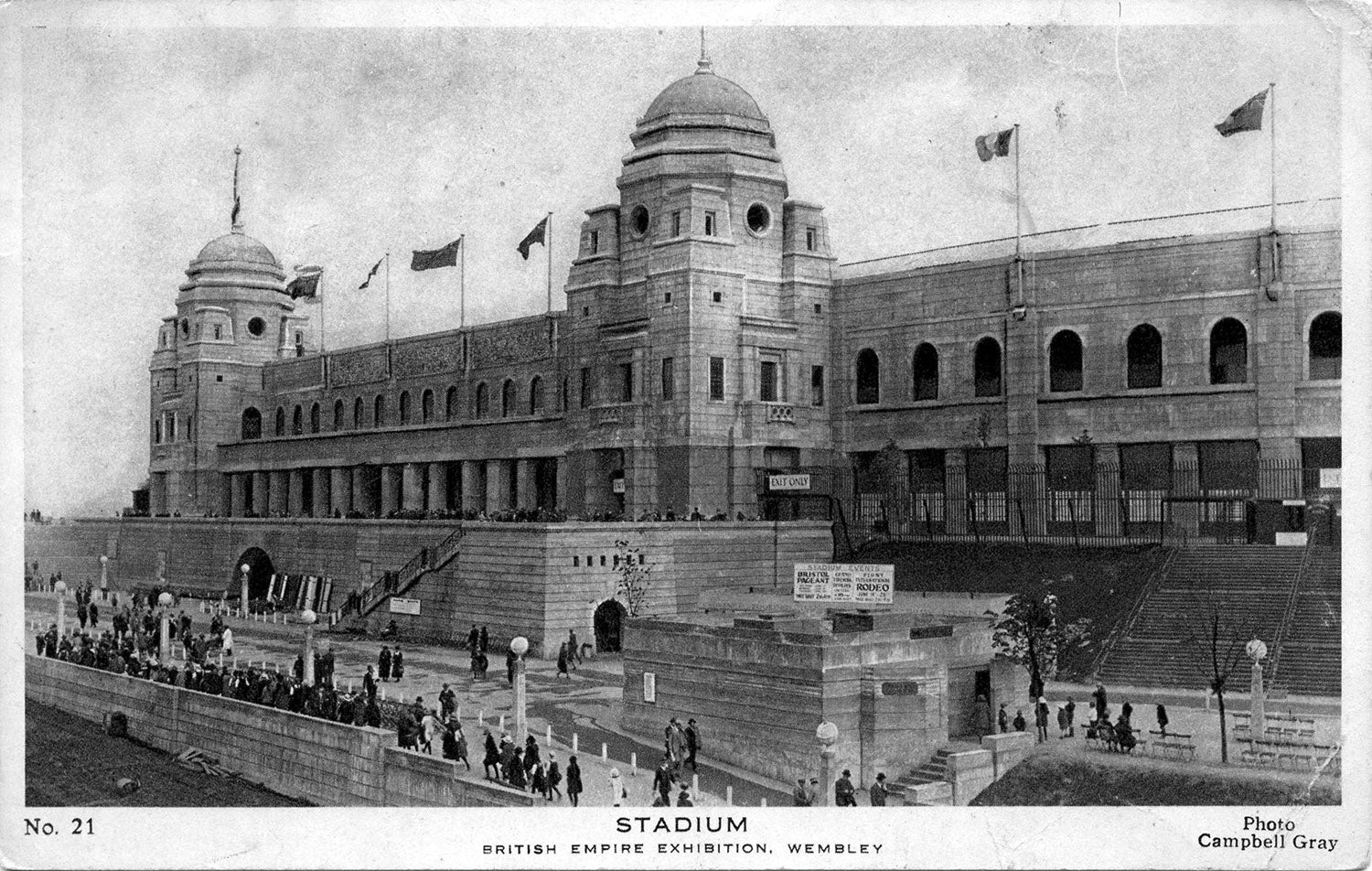This black-and-white photograph, reminiscent of an old postcard, captures Wembley Stadium during the British Empire Exhibition. The grand, multi-level stone building prominently features two dome-topped towers with mini-towers at each corner. The structure's first level is supported by numerous rectangular stone pillars, while the second level showcases large archways. At the top, several flags wave, hinting at a breezy, overcast day. Below, a considerable crowd is gathered, filing into the stadium and ascending a staircase that leads inside. The bottom of the image displays the text: "NO.21" on the left, "Stadium" in the center, followed by "British Empire Exhibition, Wembley," and "Photo Campbell Gray" on the right. Amidst the crowd, trees, benches, and lampposts can be seen, adding to the scene's historical ambiance.